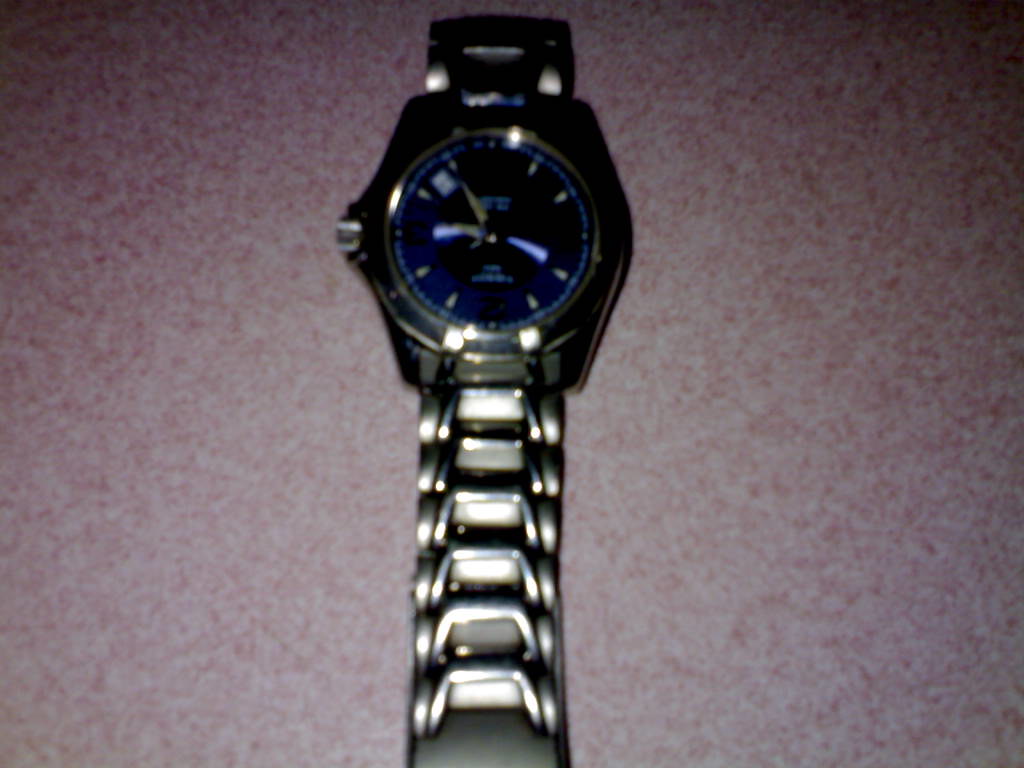In a dimly lit indoor setting, the photograph captures a wristwatch that is the focal point, highlighted by the camera's flash. The background surface, speckled in red and white hues, adds a vibrant contrast to the scene. At the center sits the elegant timepiece, predominantly constructed of silver metal. The wristwatch features a sleek silver metal band, while its face is an eye-catching blue. The watch face displays silver hour and minute hands, along with a blue-illuminated second hand. Tiny silver notches mark the hours, and subtle silver inscriptions grace the background of the watch face. The watch boasts additional silver elements, including a side dial, completing its sophisticated design.